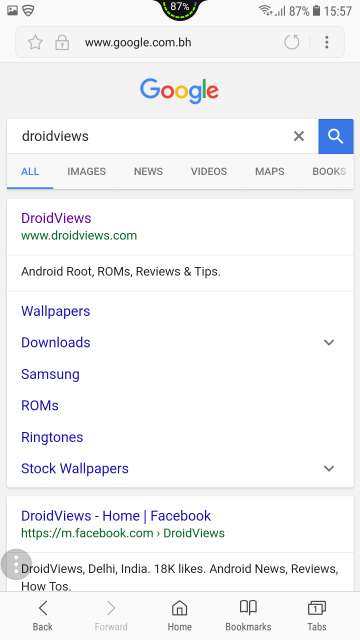This is a detailed screenshot of a Google search on a mobile phone, displaying the search results page for 'Droid Views'. At the top, the URL is www.google.com.bh, indicating the Bahrain version of Google. To the left of the URL, there's a star icon for bookmarking, followed by a lock icon symbolizing a secure connection, a refresh icon, and the three-dot menu for additional options. The background features a gradient of pale gray and white.

Beneath this, the iconic multi-colored Google logo is prominently displayed above the search bar. The query 'Droid Views' appears in the search field, with a magnifying glass icon enclosed in a blue block on the far right. Below the search bar, navigation options 'ALL', 'IMAGES', 'NEWS', 'VIDEOS', 'MAPS', and 'BOOKS' are listed horizontally in all caps.

The first search result is highlighted within a white box. The text 'Droid Views' is shown in purple, indicating a previously visited link. Directly below in dark green text is the URL www.droidviews.com. Additional descriptive text includes 'Android Root, ROMs, Reviews, and Tips'. A menu for Droid Views is also visible within the same box, featuring options such as 'Wallpapers', 'Downloads', 'Samsung', 'ROMs', 'Ringtones', and 'Stock Wallpapers'.

The second search result titles 'Droid Views-Home-Facebook' and contains information about the Droid Views Facebook page, noting 'Droid Views, Delhi, India, 18,000 Likes, Android News, Reviews, How-To's'.

At the bottom of the screen, the phone's navigation menu is displayed with back and forward arrows, a home icon, bookmarks, and tabs options, all arranged horizontally.